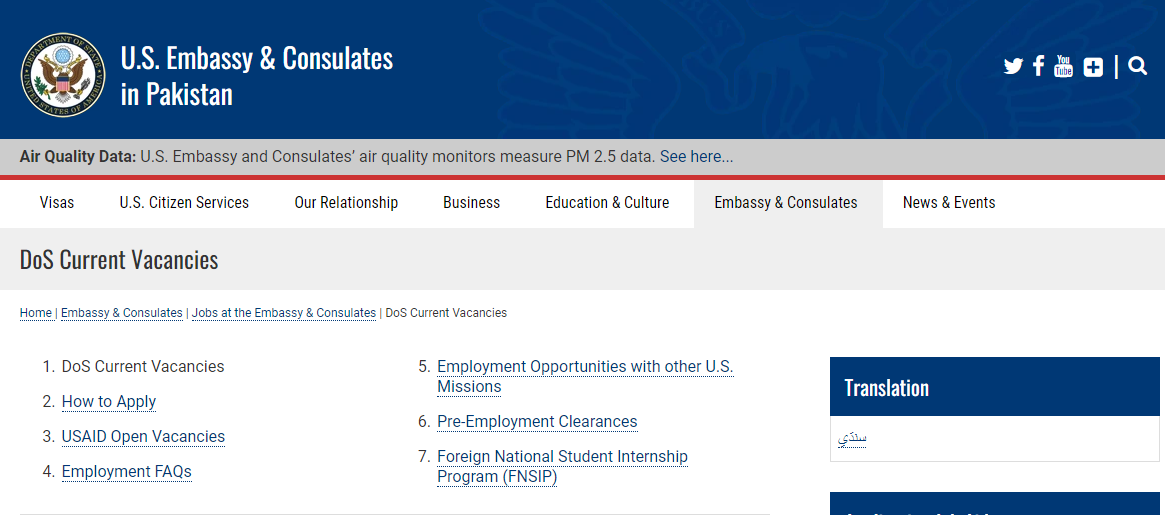This image captures the interface of a desktop application designed for the U.S. Embassy and Consulates in Pakistan. Dominating the top left corner is the emblem of the United States government featuring a bald eagle, clutching a wreath of peace with one talon and arrows with the other, symbolizing the nation's capacity for both peace and war.

Adjacent to the emblem are social media shortcuts for Twitter, Facebook, and YouTube, separated by a vertical line and followed by a magnifying glass icon representing a search function. The interface boasts a predominantly blue background with white text. Below the emblem, a prompt displays "Air Quality Data" along with a description that reads, "The U.S. Embassy and Consulates air quality monitors measure PM 2.5 data," which also includes a hyperlink inviting further exploration.

A red line runs horizontally across the screen, segmenting the interface into various navigational tabs labeled: "Visas," "U.S. Citizen Services," "Our Relationship," "Business," "Education and Culture," "Embassy and Consulates," and "News and Events." The "Embassy and Consulates" tab is currently selected, revealing sub-options and a detailed list beneath.

Within the "Embassy and Consulates" section, users find the title "DOS Current Vacancies." The navigation bar, situated below a secondary red line, includes links such as "Home," "Embassy and Consulates," "Jobs at the Embassy and Consulates," and "DOS Current Vacancies." The selected "DOS Current Vacancies" category presents a detailed list as follows:

1. DOS Current Vacancies
2. How to Apply
3. U.S. Aid Open Vacancies
4. Employment FAQs
5. Employment Opportunities with Other U.S. Missions
6. Pre-Employment Clearances
7. Foreign National Student Internship Program (FNSIP)

To the right, there is a section marked "Translation," featuring a blue background with white font, aimed at providing language assistance, enhancing the accessibility and user-friendliness of the application.